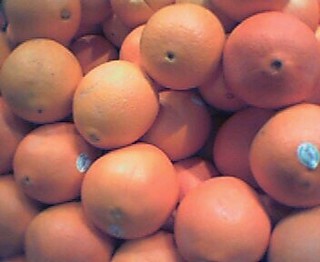This is an overhead view of a pile of oranges, possibly contained within a basket or box, filling the frame entirely. The focus is slightly off, but the fruit can be identified by their orange color and the tips where the stems used to be. There are about 25 oranges, some of which are ripe and vibrant, while others show signs of wear, discoloration, and rough texture. Among them, three randomly placed oranges feature small white stickers with black lettering. The lighting, coming from the top of the image, casts shadows on the fruit, providing some depth despite the muted colors and slight out-of-focus capture. There's a mix of deep orange, pale orange, and some with traces of green, indicating varying degrees of ripeness. The scene is tightly framed, focusing solely on the oranges without showing the surrounding area or container.